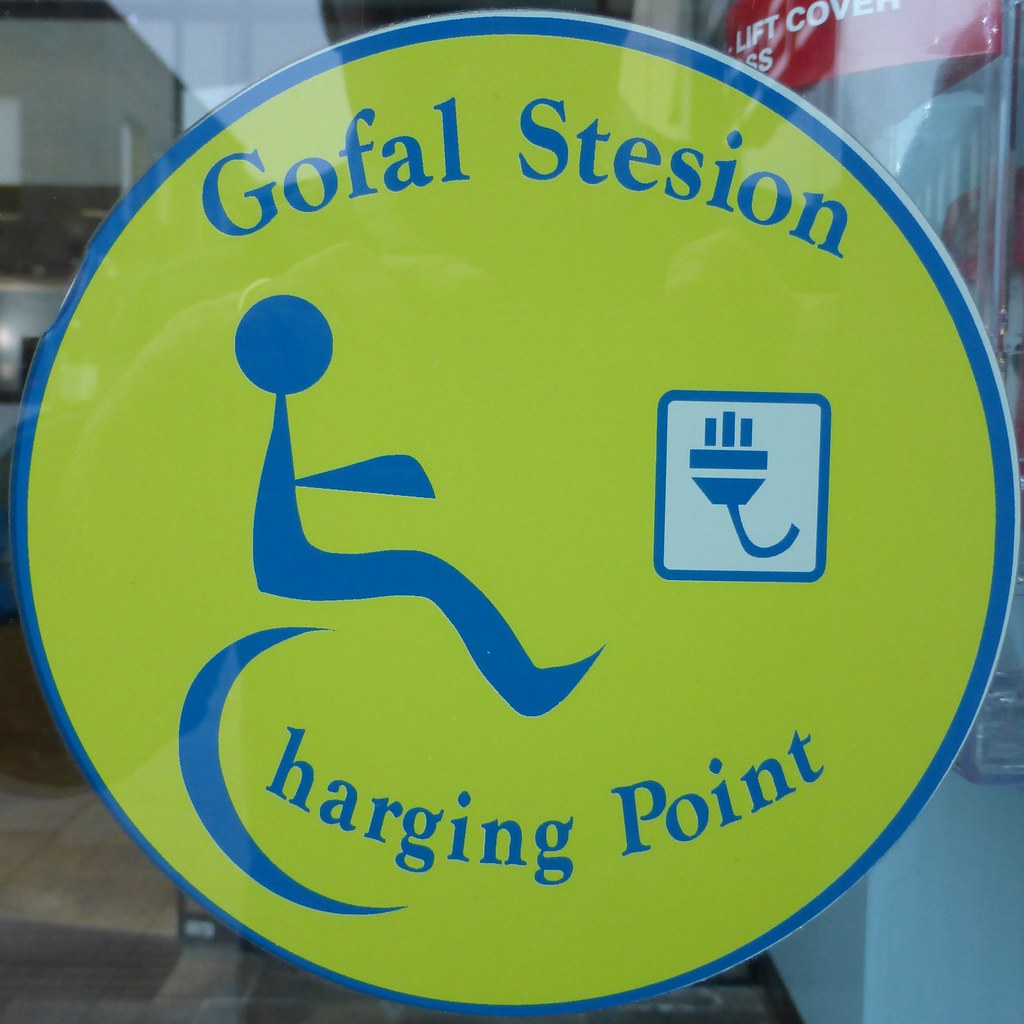This is a square color photograph featuring a close-up of a circular sign positioned behind an exceptionally clean window, likely reflecting an office space in the background. The sign, which nearly occupies the entire photo, is predominantly bright yellow with a blue border around its edge. Inside the circle, there's blue text, "G-O-F-A-L-S-T-E-S-I-O-N" at the top and "Charging Point" at the bottom. The center is split between two graphics: on the left, an image resembling a person seated, possibly in a wheelchair, forms a stylized letter 'C' for "Charging Point," and on the right, a small blue square contains an illustration of an electrical plug. The combination of elements suggests that the sign designates a charging point, possibly for electric mobility devices like wheelchairs.